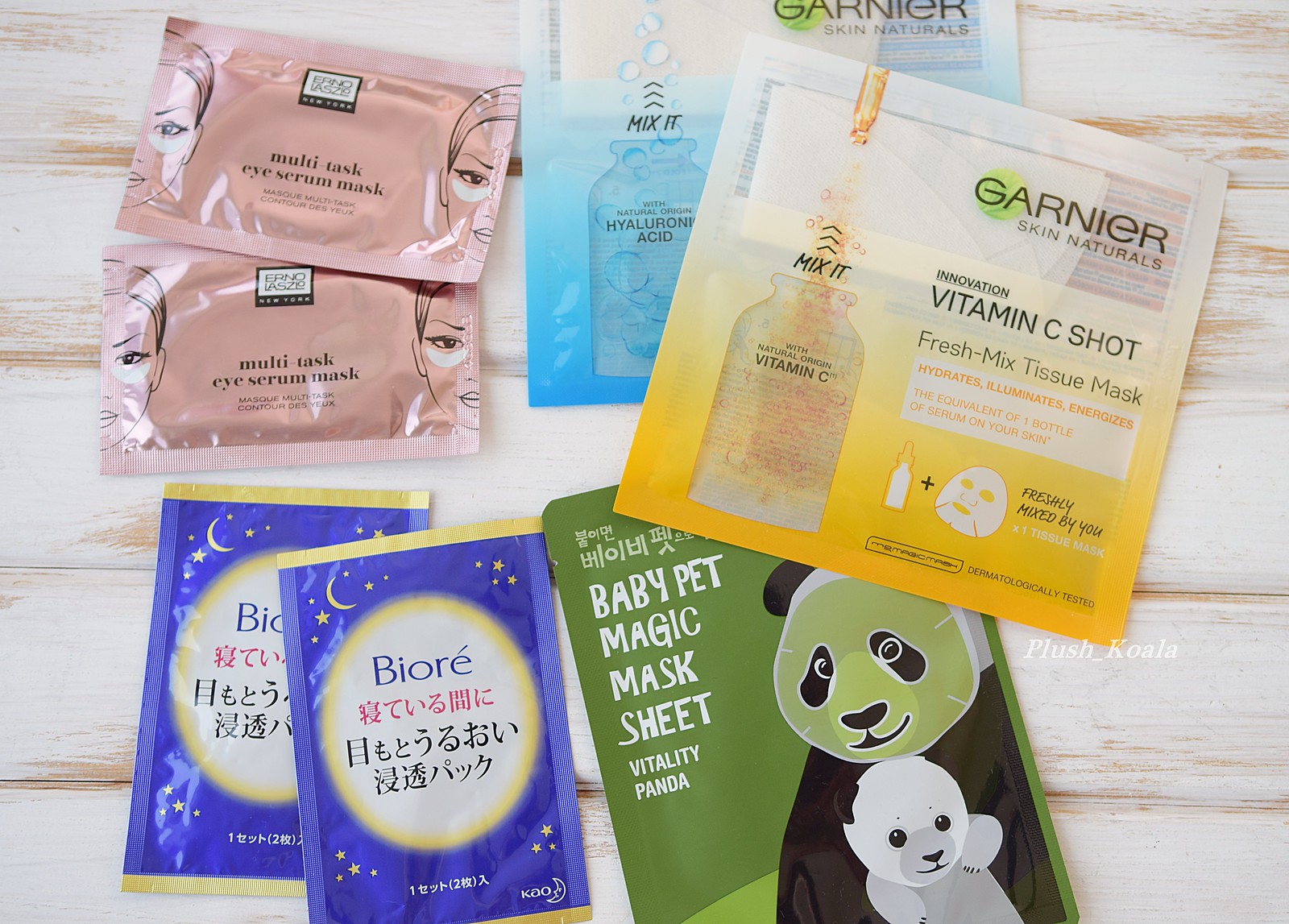This is an image displaying an assortment of single-use sheet masks arranged on a white wooden surface. 

- In the top-left corner, there are two rose gold packages featuring a design of half a woman's face with under-eye pads. The packaging is labeled "Erno Laszlo New York Multitask Eye Serum Mask."

- To the right, there are two Garnier Skin Naturals masks. The top mask has a yellow package labeled "Mix It with Natural Origin Vitamin C," and the blue package beneath it states, "Mix It with Natural Origin Hyaluronic Acid." Both promote an innovative concept of freshly mixed tissue masks that hydrate, illuminate, and energize the skin, equivalent to a full bottle of serum.

- Below the Garnier masks is a green package illustrated with a panda bear wearing a green mask while holding a baby panda. The package bears some Korean text at the top and is labeled in white text as "Baby Pet Magic Mask Sheet Vitality Panda."

- To the left of the green package are two Biore masks with gold trim and a purple-blue background adorned with yellow stars and moons. An oval with a yellow border in the center bears the Biore logo and some text in various languages.

The detailed arrangement and vibrant packaging of these masks provide a rich visual summary of diverse skincare options.